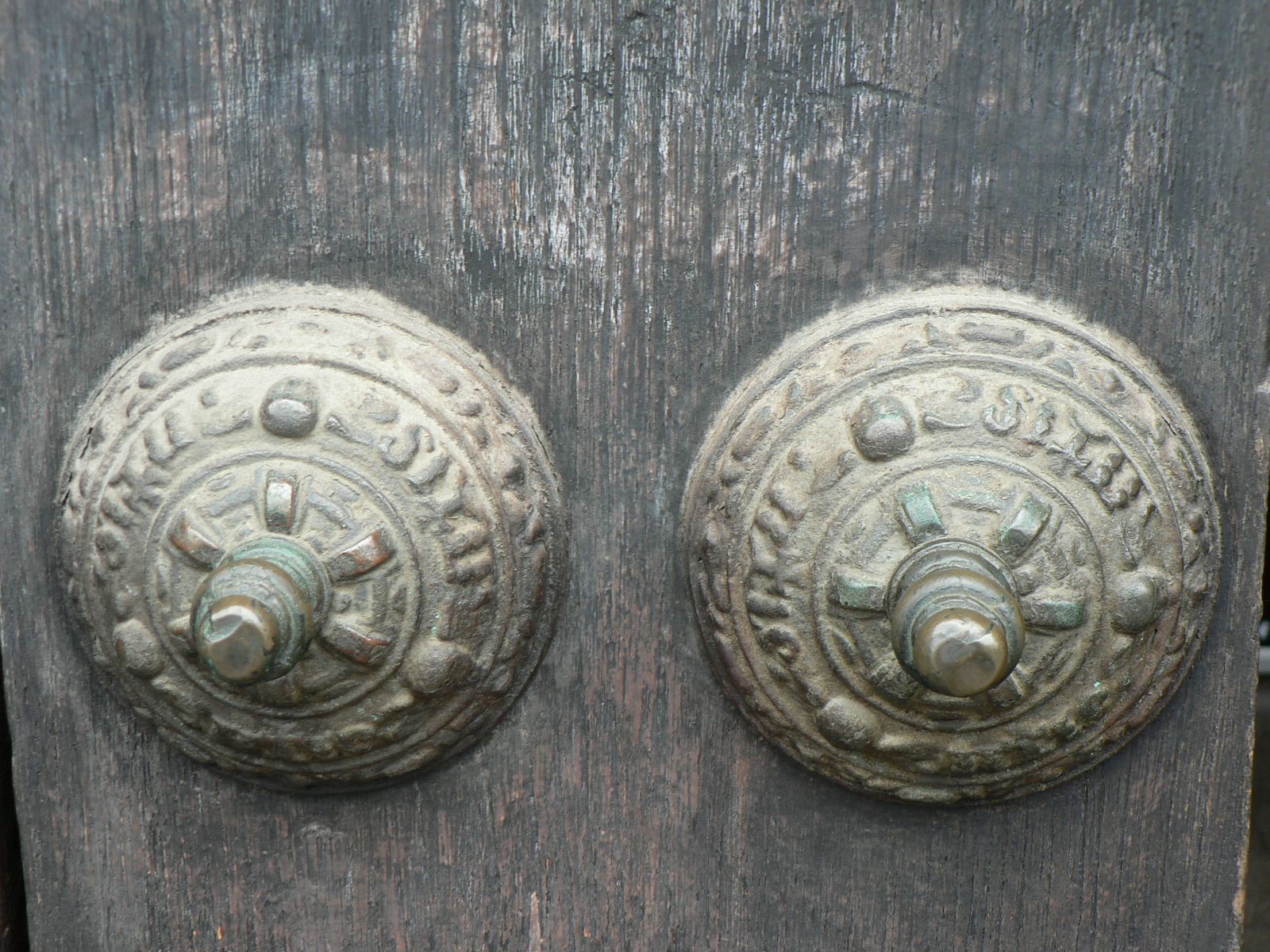The photograph features two identical, weathered metal discs on either side of the image, mounted on a vertical piece of dark-toned, worn wood streaked with white and brown. The discs, likely made of iron or cast iron given the visible grain, boast an intricate design. Each consists of multiple decorative rings: an abstract outer pattern of ovals and circles, followed by a strip with faint, weathered text, most likely Latin. Situated in the innermost section are smaller circular patterns, with each disc displaying a unique arrangement of these circles at varying angles. 

At the center of each disc, six rectangular bulges form a flower-like shape, culminating in a large, silver-finished knob resembling a bolt or screw. These knobs, adorned with additional delicate decorations, have a greenish tint on the top, indicating age. The entire setup exudes an air of antiquity, although their exact purpose remains a mystery; they might be decorative elements or perhaps functional components such as vintage doorbells.